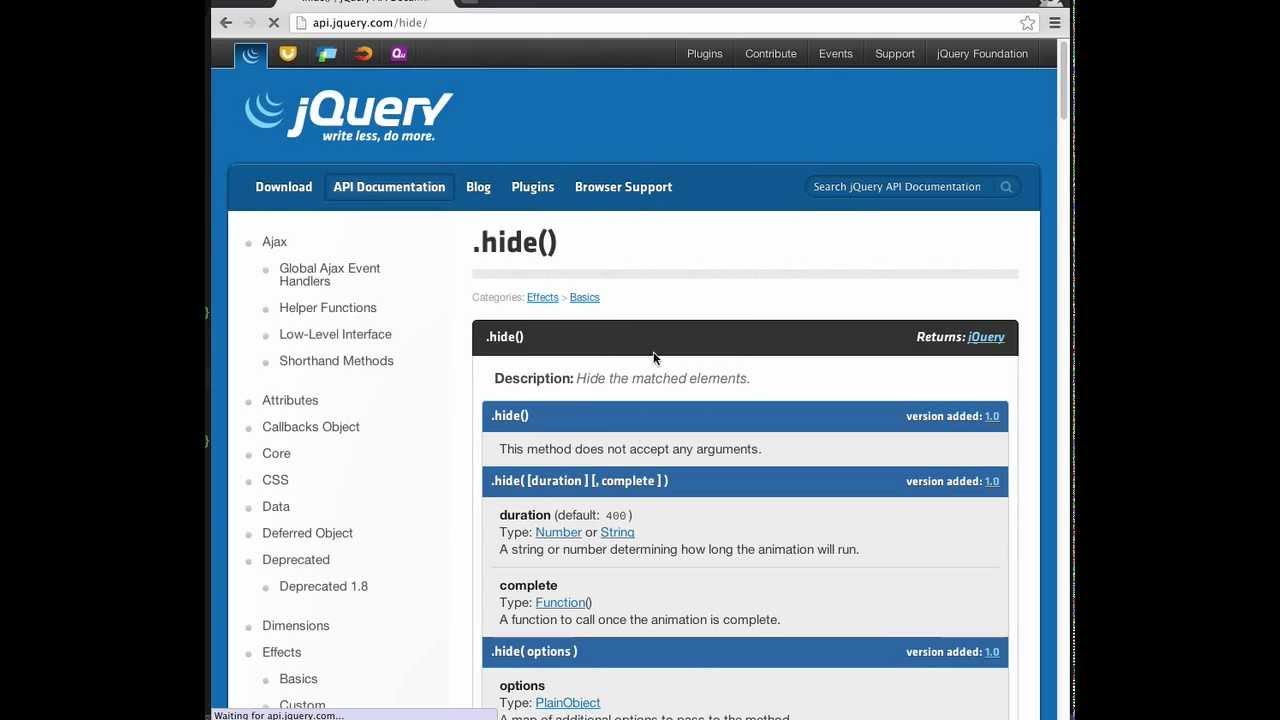The image is a screenshot taken from a web page displayed inside a web browser with a single tab open. The browser's address bar shows the URL: "api.jquery.com/hide/". The screenshot is placed against a black backdrop, which is visible along its left and right edges. The web page features a somewhat dated design style with a prominent blue header displaying the jQuery logo and the slogan, "write less, do more."

At the very top of the page, there is a black navigation bar with buttons labeled: Plugin, Contribute, Events, Support, and jQuery Foundation. The main content of the screenshot is dedicated to API documentation for the jQuery method, `.hide()`. This section provides detailed information on how to implement the `.hide()` method within the jQuery library, illustrating its practical use cases and applications in web development.